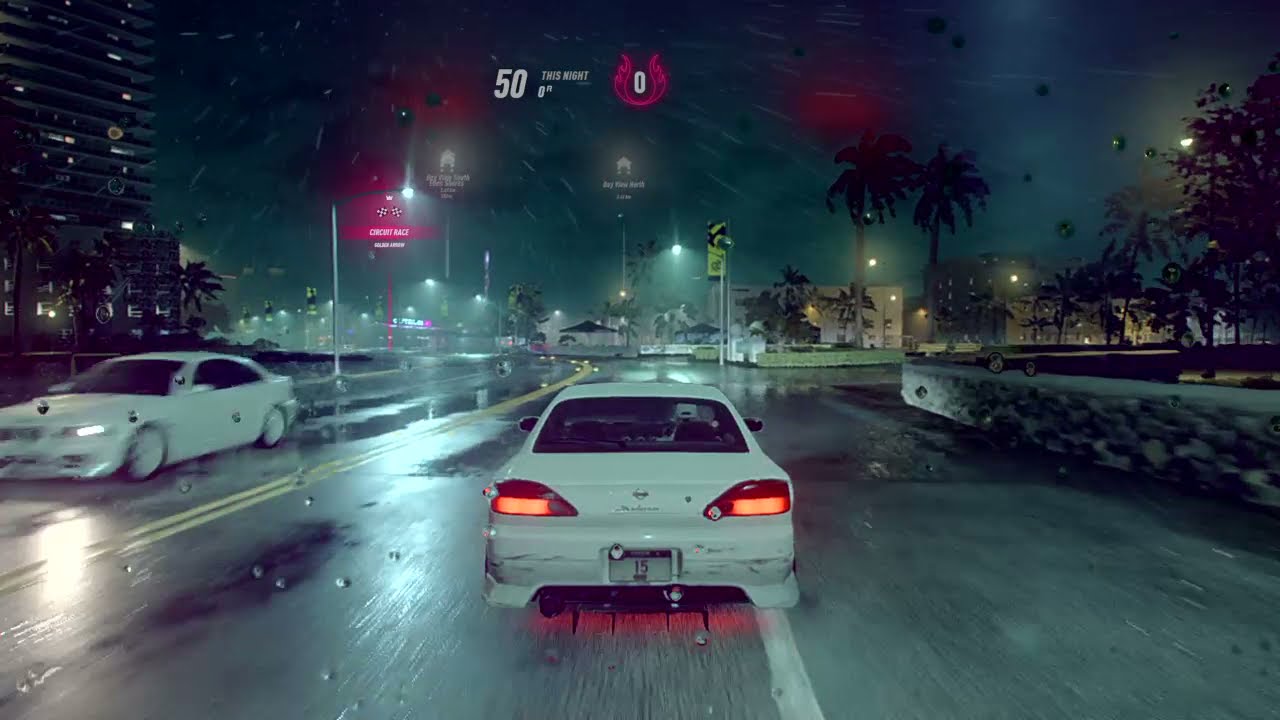This nighttime scene, possibly from a video game or digitally enhanced photograph, captures a wet and rainy highway with a dynamic, almost speed-blurred effect. The vantage point is from a moving vehicle in the right-hand lane, immediately behind a white car with its red taillights illuminated. On the opposite side of the blurred, rain-streaked road, another white car approaches with bright white headlights. The road, shiny and slick under the rain, curves to the left, lined by yellow dividing lines and bordered by white side markings. Multi-story apartment and high-rise buildings flank the left side, with more buildings in the distance on the right. Palm trees and city lights add to the urban setting. Rain is pouring down, with droplets visible against the dark sky and on the camera lens. The image also features red and white writing along the top, which could either be highway signs or embedded graphics.